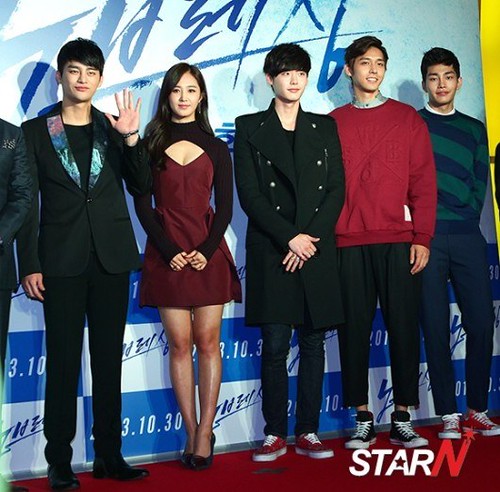This promotional image features a group of five young Asian individuals, possibly Korean entertainers such as movie stars or singers, standing on a red carpet. They are positioned in a line against a white and blue graphic backdrop, which includes illegible lettering and a checkerboard pattern towards the bottom. In the lower right-hand corner of the backdrop, the word "star" is written in white with a red star inside the 'A', followed by the letter 'N' in red with a small star at the top of the right side.

From left to right, the first individual is a man wearing a black suit jacket with colorful lapels who is raising his right hand in a wave. Next, there is a woman in a short burgundy dress with a V-cut neckline, complemented by a black long-sleeved shrug, and she has long hair worn down. The person at the center appears androgynous, likely male, dressed in a long black coat, skinny black jeans, and red sneakers. To their right is another man in a dark red pullover and black pants with black sneakers. Finally, the man on the far right is wearing a dark blue and green striped sweater paired with dark pants and red sneakers. The overall color scheme of their outfits primarily consists of blacks and reds, with some elements of green.